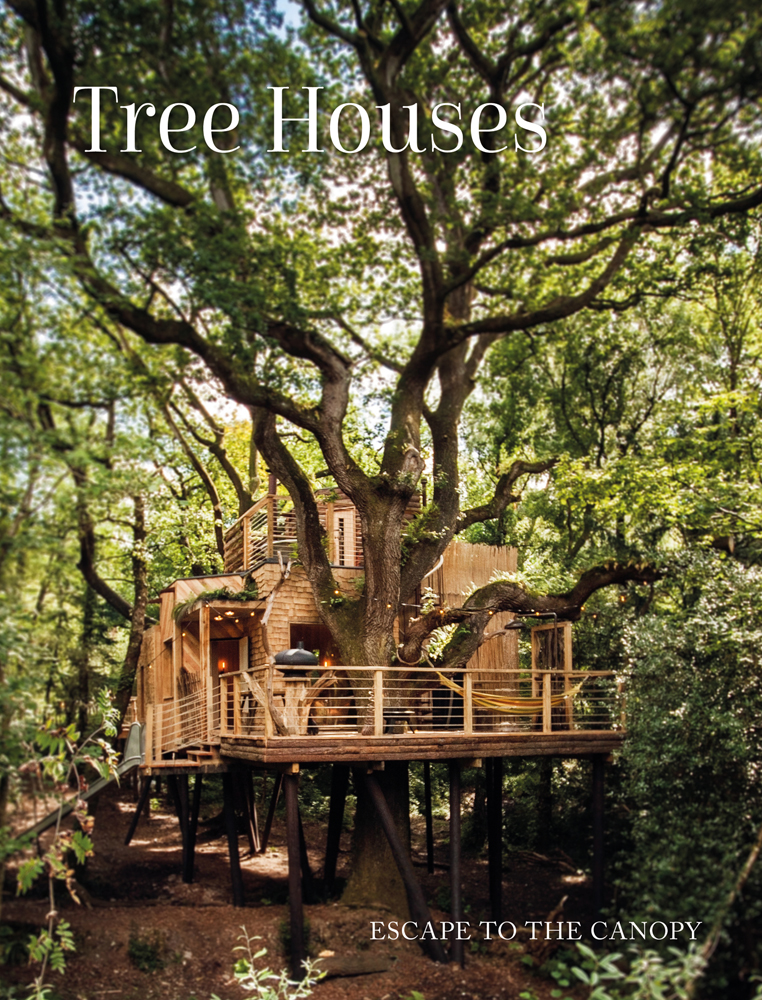This photograph captures a charming treehouse nestled in a lush, green forest. The image prominently features a majestic tree with twisty branches and green leaves, around which the treehouse is built. The house is made of warm-colored, light wood with wood shingles and is elevated off the forest floor by dark wooden stilts. A wooden porch or deck, surrounded by fencing, wraps around the front and left side of the structure. 

Notably, a hammock is seen hanging from a tree branch to the right of the house, providing a cozy resting spot. Additionally, a black round barbecue grill is positioned on the left side of the porch. The tree trunk grows through an opening in the house, emphasizing the harmonious blend of nature and architecture. 

Above the scene, in large white text, the word "treehouses" is displayed. Meanwhile, at the bottom right of the photograph, in smaller white text, the phrase "escape to the canopy" invites viewers to imagine a serene retreat amidst the trees. The photograph hints at a blue sky peeking through the canopy, adding to the idyllic atmosphere.